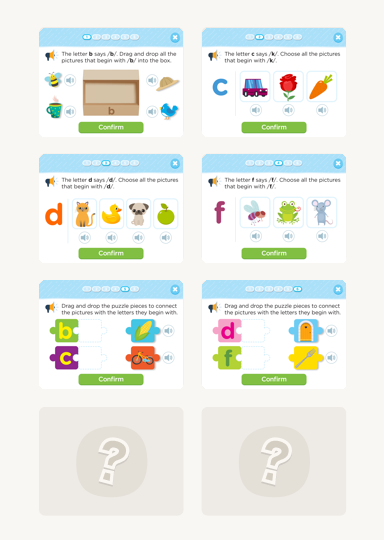This image is a tablet screenshot of an educational app designed for children. The screen displays six different sections, each containing a distinct quiz or activity. These sections are numbered consecutively from 1 to 6, with corresponding bubbles at the top that highlight the current question number.

The focus of the image is on a quiz related to phonetics and letter recognition, specifically the letter "D." The quiz instructs the user to identify all the images that start with the letter "D." The screen shows the lowercase letter "d" alongside the phonetic symbol or IPA representation to aid pronunciation. There are four illustrated options: a cat, a duck, a dog, and an apple. Below each image is an audio icon button that reads out the option when pressed, aiding auditory learning.

After the user has selected their answers, they can confirm their choices by pressing a green button labeled "Confirm." Additionally, there are two empty sections at the bottom with question marks, indicating that these questions are either yet to be unlocked or are placeholders for future content. The layout is structured into two rows and two columns, though only three sections in each column currently contain quiz questions.